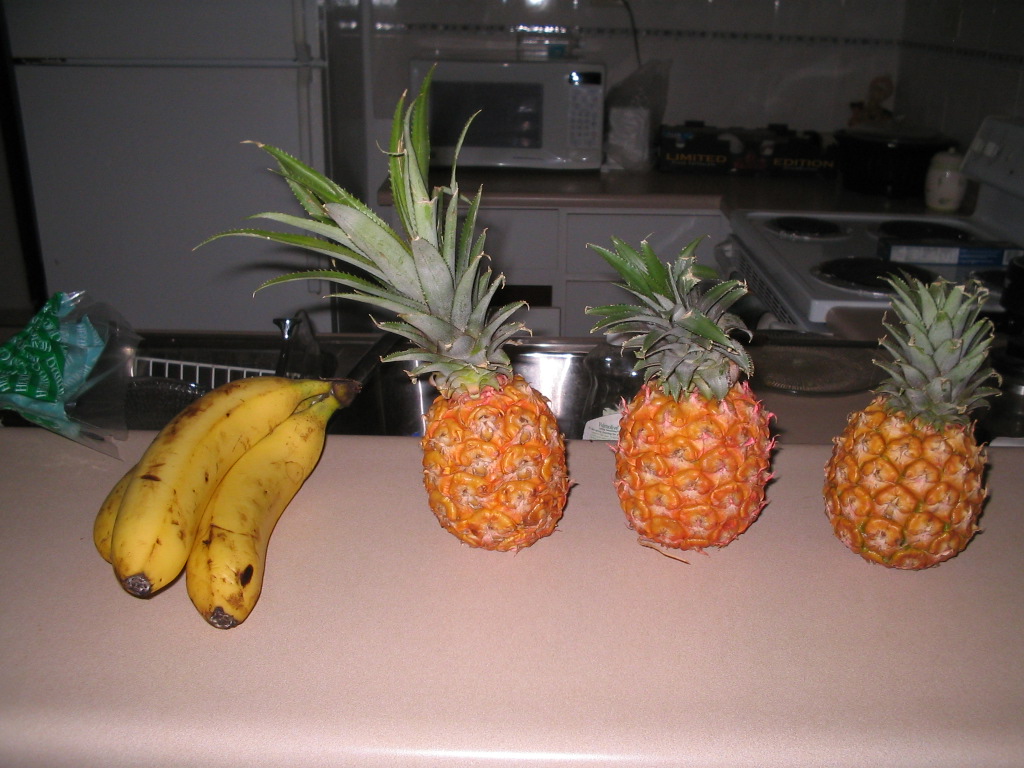This image offers a bird’s-eye view of a kitchen, taken from a slightly elevated angle that provides a comprehensive perspective without being directly overhead. Situated to the left, a plain white refrigerator anchors the scene. Adjacent to it on the right, a white microwave rests casually on the beige countertop, not built into the cabinetry. 

The countertop is dotted with various items, contributing to the lived-in feeling of the space. A white stove, prominently positioned, features a couple of dishrags draped over its oven handle, suggesting recent use. Near the burners, a box of some kind is visible, adding to the casual clutter of everyday life. Central to the view is a stainless steel sink equipped with a white drying rack, hinting at recent dishwashing activity.

Adding color and texture, the countertop holds an assortment of fruit: three pineapples, one with notably longer leaves than the others, and a trio of bananas speckled with brown spots. The scene is softly illuminated by ambient light, casting varied shadows across the neutral-hued surface, which enhances the depth and dimension of the image.